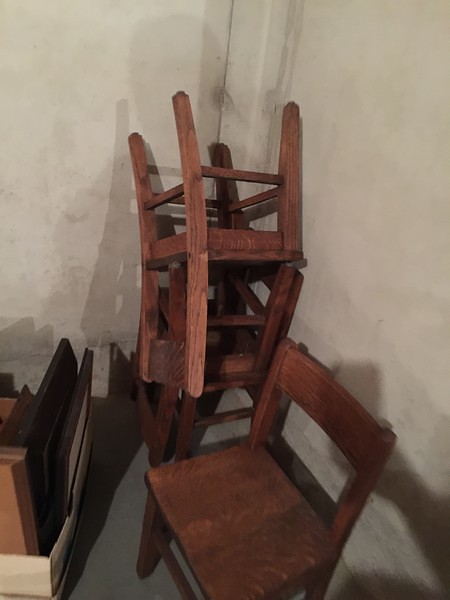This indoor color photograph captures a quiet corner of a room with an off-white wall as a backdrop. The primary subjects are several wooden chairs with a natural finish, showcasing a simplistic design. In the foreground, one chair stands alone, its back to the wall, ready for use. In the corner, three other chairs are stacked neatly; the top chair is upside down and slightly tilted, adding a touch of asymmetry. To the lower left of the image, there is a box filled with a collection of picture frames, their backs facing out. The floor beneath is light gray, and there is noticeable shadowing on the right side of the image, indicating that the light source is coming from the left. The photograph, devoid of any text or prints, is slightly out of focus, lending it a subtle, dreamlike quality.